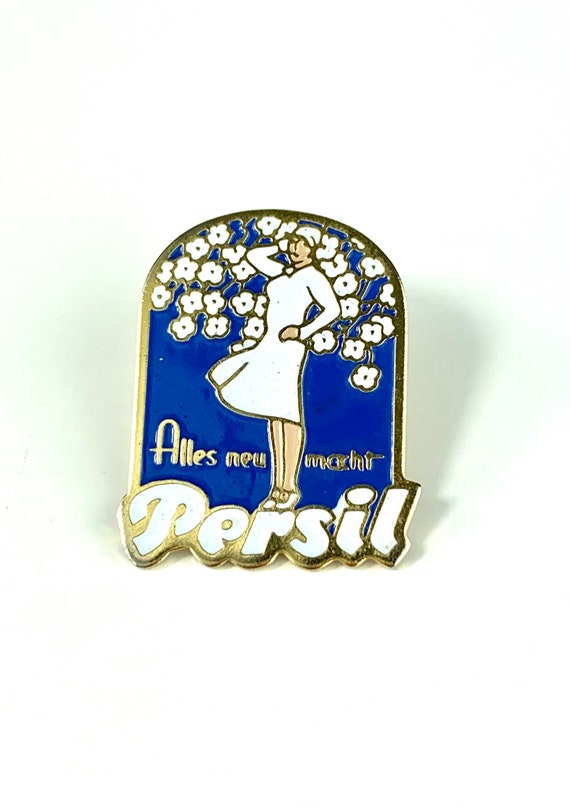This close-up photo reveals a detailed image of a pendant that resembles the top of an old-style light bulb or a half-oval shaped metal pin. The pendant features a woman with olive skin, dressed entirely in white—a long-sleeve dress, white pumps, and a white cap. With her left hand on her hip and her right hand holding her head, she stands against a royal blue background adorned with scattered white flowers. At her feet, in gold letters, is an inscription that appears to read "A-L-L-E-S N-E-U," with the remainder obscured on the right side. Below this, in distinct white text with golden embroidery, is the word "PERSIL."